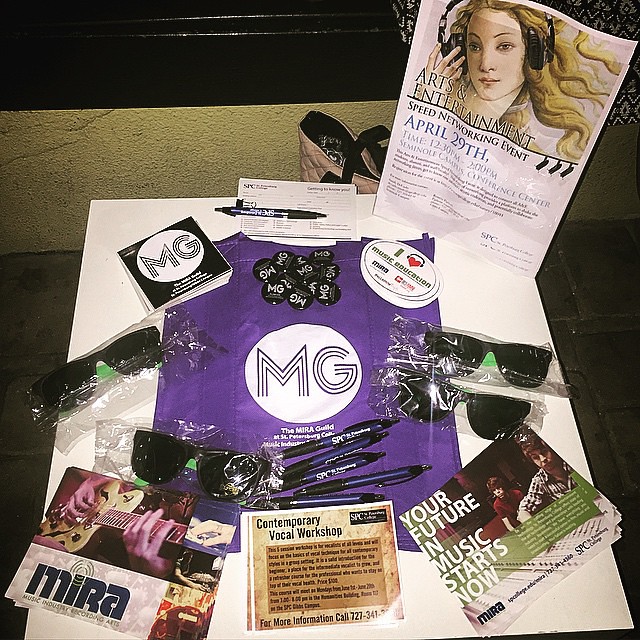The image showcases a meticulously arranged display on a white surface, possibly a table or floor, set against a rectangular gray stone backdrop. Dominating the upper right is an upright white pamphlet titled "Arts and Entertainment Speed Networking Event, April 29th," featuring artwork of a woman with blonde, curly, wavy hair wearing headphones. Beneath this pamphlet lies a collection of promotional materials: 

- A central purple bag adorned with a white circle bearing the letters MG in gray, with each letter formed by three lines.
- Several black Wayfarer sunglasses in plastic bags, equipped with green ear clips.
- A pile of black and white MG buttons.
- Various pens scattered across the display.
- Business cards and cutouts advertising "M.I.R.A. Music Recording Arts," "Contemporary Vocal Workshop," and "Your Future in Music Starts Now."
- MG-branded stickers or magnets.

These items collectively promote what's likely an MG event or program, emphasizing the arts, music recording, and opportunities in contemporary vocal training.